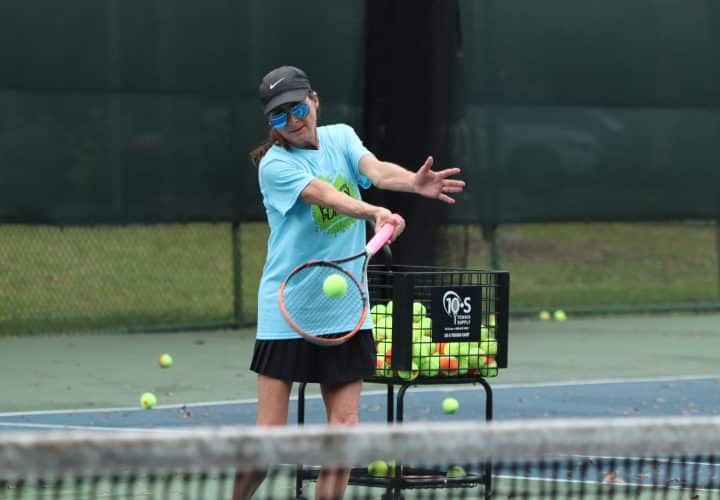The image features a woman playing tennis, captured mid-swing. She is centered in the frame, wearing a black baseball cap with a white Nike logo on the front, and round blue sunglasses. Her light blue t-shirt with short sleeves displays a green tennis ball graphic with black text inside, and she pairs this with a black skirt. Her brown hair is tied back in a ponytail. In her right hand, she grips a tennis racket with a pink handle, and she appears to be hitting a tennis ball. Her left arm is extended out to the side in a somewhat unusual position. To her left, there is a black cart filled with tennis balls, resembling a grocery cart. In the background, a tennis net with a white top border and black netting is visible, along with a fence with black poles and some grass. Several tennis balls are scattered on the ground, suggesting she might be practicing her swings.